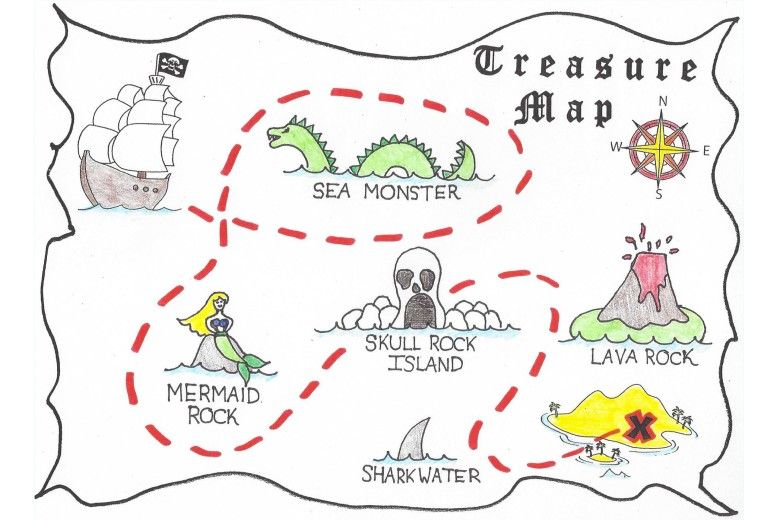This is a childlike illustration of a treasure map featuring a worn and weathered parchment appearance. The rectangular map has irregular, curvy edges, reminiscent of a motion-blown flag. Prominently, in the upper right corner, calligraphic script spells out "Treasure Map," accompanied by a compass. The map is dotted with various labeled landmarks and vivid drawings. In the upper left corner, a brown pirate ship flies a black Jolly Roger flag atop its mast and is depicted with numerous full white sails. A red dashed line representing the treasure trail meanders from this ship across the map, ultimately leading to a yellow sandy beach adorned with palm trees and an 'X,' marking the treasure's location in the bottom right corner.

Key features include:
- **Mermaid Rock** in the lower left corner, showing a mermaid with long blonde hair sitting on a rock amidst ocean waves.
- A **green sea monster**, resembling the Loch Ness Monster, floating in the central part of the map, labeled “SEA MONSTER” in all-capital black letters.
- **Skull Rock Island** noted below the Sea Monster, followed by an area labeled “SHARK WATER,” indicating shark-infested waters.
- To the far right is **Lava Rock**, depicted as an erupting volcano.

This vibrantly colored map is filled with fantastical details that animate its adventurous theme, from mythical creatures to perilous terrains.